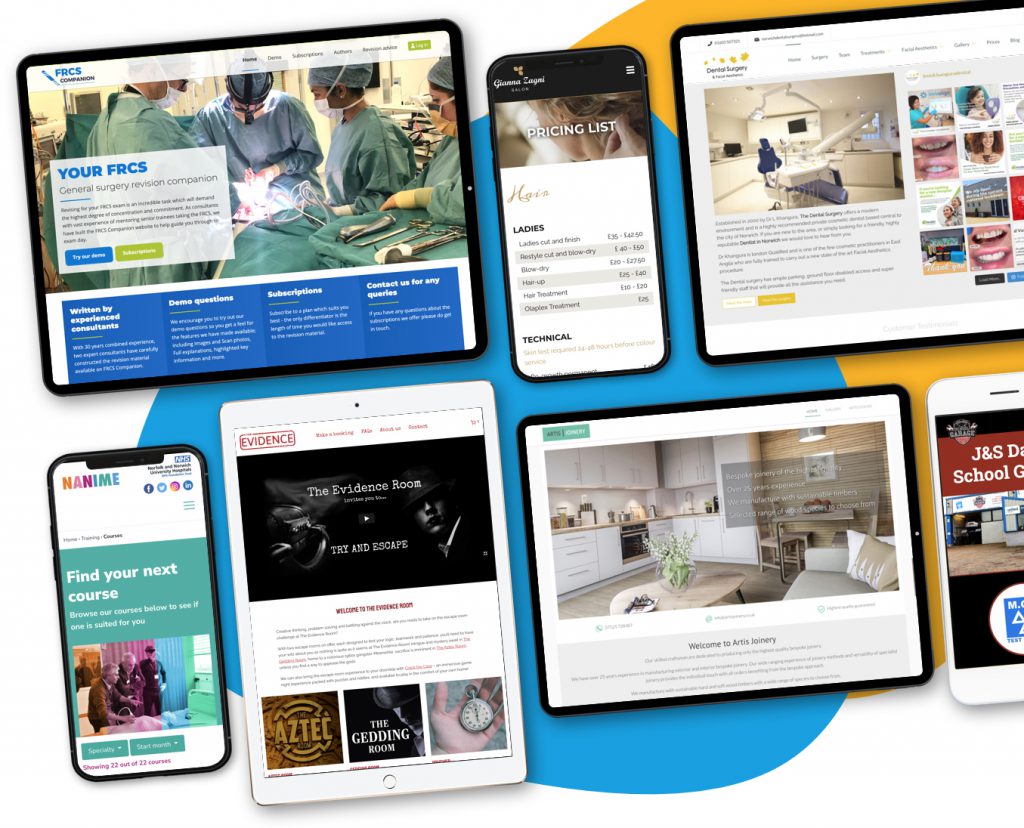The image features a colorful background with a large blue circle on the left side and an equally large orange circle on the right. Overlaying this vibrant backdrop are several distinct boxes, each containing different images and text.

In the top-left corner, there's a tablet displaying a photo of doctors working in surgery. This tablet screen is crowded with various boxes and writing, providing additional context or information related to the medical scene.

To the right of this, there is an image of a black smartphone. On the phone's screen, the text "Pricing List" is prominently featured in white, along with the words "Ladies and Technical" in black writing.

Further to the right, another tablet is shown with a dentist office visible on its screen. This device's display includes pictures of people, along with detailed images of mouths and teeth, indicating a focus on dental care.

Beneath these is a large tablet screen with the title "The Evidence Room" and a prompt to "try and escape." This main tablet screen is accompanied by three smaller sections: one says "Aztec," another reads "The Getting Room," and the last features an image of a hand holding a stopwatch.

To the left of this central tablet, there's another image of a smartphone. The phone screen showcases a website with the headline "Find Your Next Course" in white text against a blue background. Below this text, there’s a picture of three men standing side by side, all pointing and looking at something off-screen.

The diverse elements in this image combine to create a visually engaging collage with themes ranging from medical and dental fields to escape rooms and educational courses.